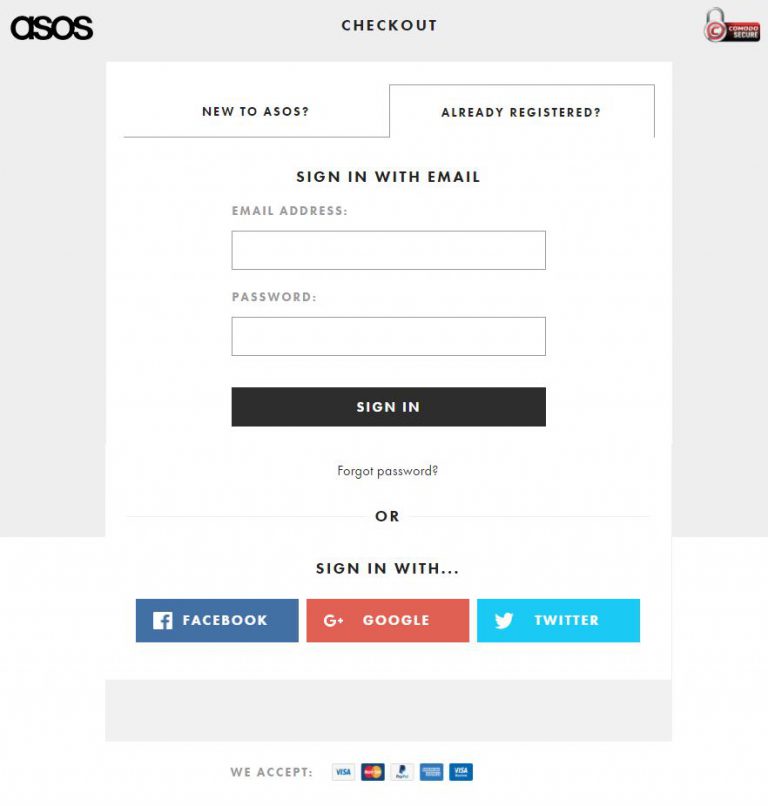The ASOS checkout page features a visually appealing design with a striking backdrop. In the upper right corner, there is an icon resembling a combination lock, symbolizing security. Next to it, a dual-colored box—red on top and black on the bottom—encases a "Checkout" label.

The central part of the page presents two prominent options: a white box labeled "New to ASOS?" and another box labeled "Already registered?" Both prompts guide users based on their status. 

At the center, bold black letters instruct users to "Sign in with email." Below this heading, there are input fields: one for the "Email address" and another for the "Password," both denoted in gray within long, gray boxes. A solid black "Sign In" button with white text is prominently displayed beneath these fields.

Further down, options are provided for account recovery and alternative sign-ins. The "Forgot password," option is noted alongside the phrase "or sign in with..." followed by three icons representing Facebook (blue), Google (red), and Twitter (light blue).

At the bottom, a gray box lists the accepted payment methods, including Visa, MasterCard, PayPal, American Express, and an unspecified icon. This section underscores ASOS's diverse payment acceptance policy.